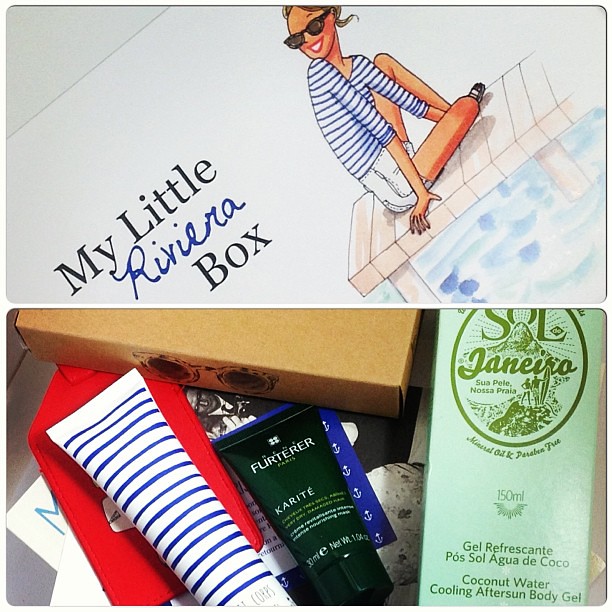This promotional image is a square format combining color illustration and photography. The top half features an illustration of a woman in a blue and white striped shirt and white shorts, sitting on a pier and smiling while looking out at the water. She is wearing sunglasses, and to her left, there is handwritten text in blue that reads "My Little Riviera Box." The bottom half showcases a photograph of the box's contents, arranged neatly. The items include a blue and white striped tube, a black tube, and a green bottle labeled "Gel Refrescante Coconut Water Cooling Aftersun Body Gel." Additionally, there is a box that reads "Genesa, mineral oil, gel refuse," and other skincare products. The overall design combines a realistic photographic style with graphic illustrations, emphasizing the holiday and beauty theme.